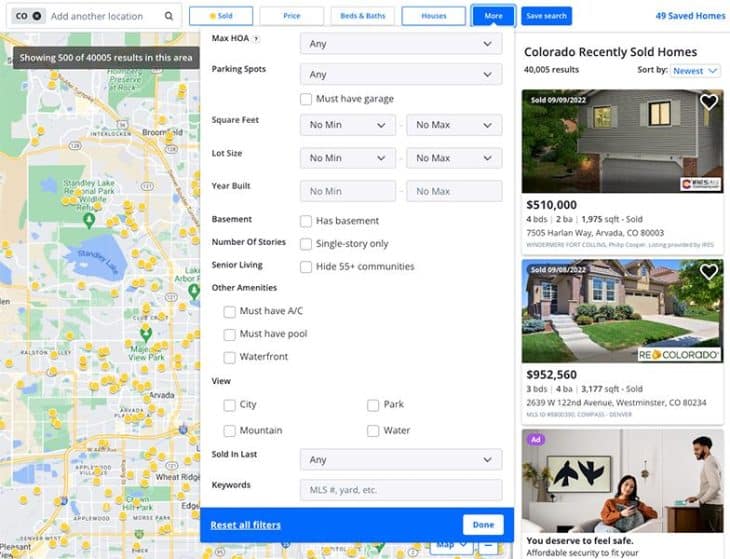A detailed Zillow property search page is displayed on a desktop site with a clean, white background. At the top, a navigation bar is featured with "CO" indicating the search is for Colorado properties. To the right, there's an option to "Add another location," followed by a search box with a magnifying glass icon. The bar also includes filters such as "Sold," "Price," "Bed and baths," "Houses," "More," and "Save search," with "Sold" highlighted in a darker blue box accompanied by a small gold medallion. "More" and "Save search" buttons are in blue boxes. 

To the far right, a hyperlink indicates "49 saved homes." Below this navigation bar, text to the left notes "Showing 540,005 results in this area," followed by a map. Centrally located below the map are additional filter options like "Max HOA," "Parking spot," "Square feet," "Lot size," "Year built," "Basement," "Number of stories," "Senior living," "Other amenities," "View," "Sold in last," and "Keywords," each with drop-down menus or checkboxes.

At the bottom of this section, a blue banner displays options to "Reset all filters" and "Done," with "Done" featured in a white box framed in blue. To the right, the page lists "Colorado recently sold homes," totaling 510,952,560, accompanied by images of the homes. Beneath this, a message states, "You deserve to feel safe. Affordable security to fit your needs," highlighted with a small blue or purple box labeled "Ad" in the upper left corner of the message.